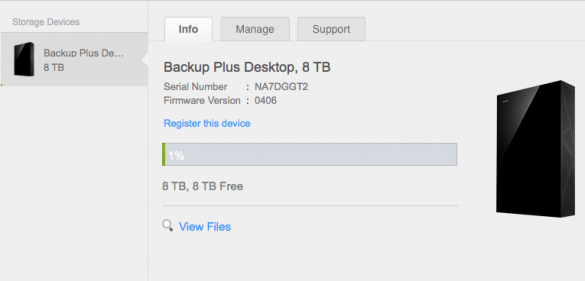This image showcases a detailed interface of a storage device management system. The layout is divided by a vertical gray line, separating it into two sections, with the right side occupying a larger portion of the screen.

On the left side, we see a dark gray rectangle featuring the title "Storage Devices." Within this section, there is a black box resembling an electronic device. The text "Backup plus DE..." is prominently displayed in black, with "DE" capitalized. Beneath this, the storage capacity is indicated as "8TB."

The right section consists of three tabs - the first tab has a white background labeled "Info" in gray text, while the other two tabs, "Manage" and "Support," have gray backgrounds. Below the tabs, detailed information about the device is presented: "Backup plus Desktop, 8TB," followed by the serial number "NA7DGGT2" and the firmware version "0406." Highlighted in blue, it states "Registered as a Device."

Further down, a gray rectangle contains a green progress bar indicating "1%." Next to it, the available capacity is detailed as "8TB free." A thin gray line separates this section from the subsequent elements, including a gray and white magnifying glass icon with the blue text "View Files."

The right section also prominently features the black electronic device box seen earlier on the left side.